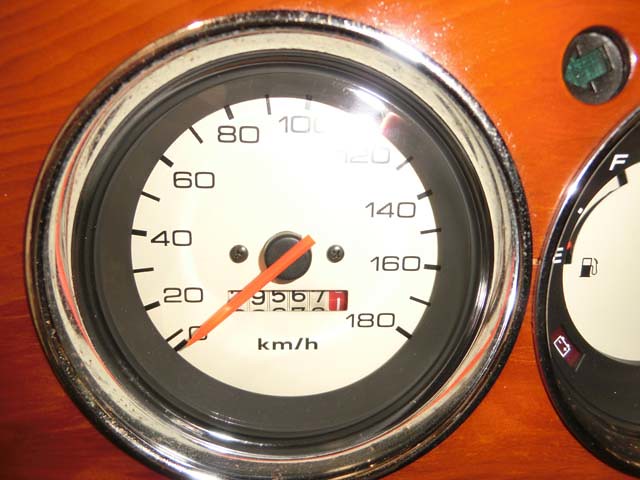This is a detailed photograph of a vintage car speedometer and gauge cluster removed from its dashboard, resting on a wooden surface. The speedometer, encased in a shiny glass cover and framed with a chrome ring and black inner frame, prominently features a classic analog display. 

The speedometer needle is positioned at zero miles per hour, with a scale that includes intervals of 20, ranging from 0 up to a maximum of 180 mph. Below the speed indicator, an old-fashioned, non-digital odometer with rolling numbers is partially visible. The odometer displays the digits 9, 5, 6, and 7, with the first numeral obscured by the speedometer needle, indicating the vehicle’s mileage. A "KM/H" inscription signifies that the speed is measured in kilometers per hour. 

To the right of the speedometer is a fragment of the fuel gauge, only revealing the left side, which includes an 'E' for empty, a gasoline pump icon, the 'F' for full, and part of the battery indicator. A small, circular indicator with a green arrow sits atop this gauge, though it appears faded and somewhat rusted. The flash of the camera introduces reflections and glare on the shiny surfaces of these vintage instruments.